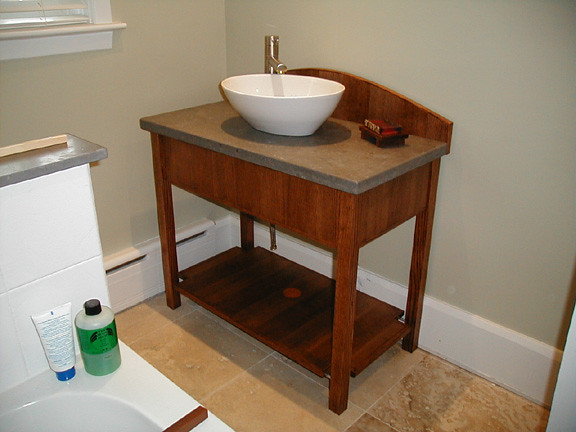The image depicts a meticulously designed bathroom showcasing a blend of warm and cool tones. The khaki-colored bathroom walls are complemented by white and tan floor baseboards, which seamlessly transition to a travertine tile floor.

A standout feature is the unique sink, mounted on a butcher block-like wooden cabinet. This cabinet boasts a low shelf near the floor and a sleek countertop area. The white sink, styled like a bowl placed on a tabletop, adds an elegant touch. To the right of the sink, there appears to be Decorative items or possibly soap, enhancing both functionality and aesthetics. The modern, minimalistic faucet with a slight curve perfectly complements the setup. The cabinet's backdrop, in a matching tan hue, also has a subtle curve, providing a cohesive look.

On the left side, there's a partial wall with a gray top, likely concealing a toilet due to its separation design. Adjacent to this partial wall, the top left corner of the bathtub is visible. Positioned on the edge of the tub are a white lotion bottle with a blue cap and blue lettering, and a cylindrical bottle with a small mouth, a black lid, and a green label containing what appears to be a yellow substance. The pristine white tub adds to the overall clean and modern aesthetic of the bathroom.